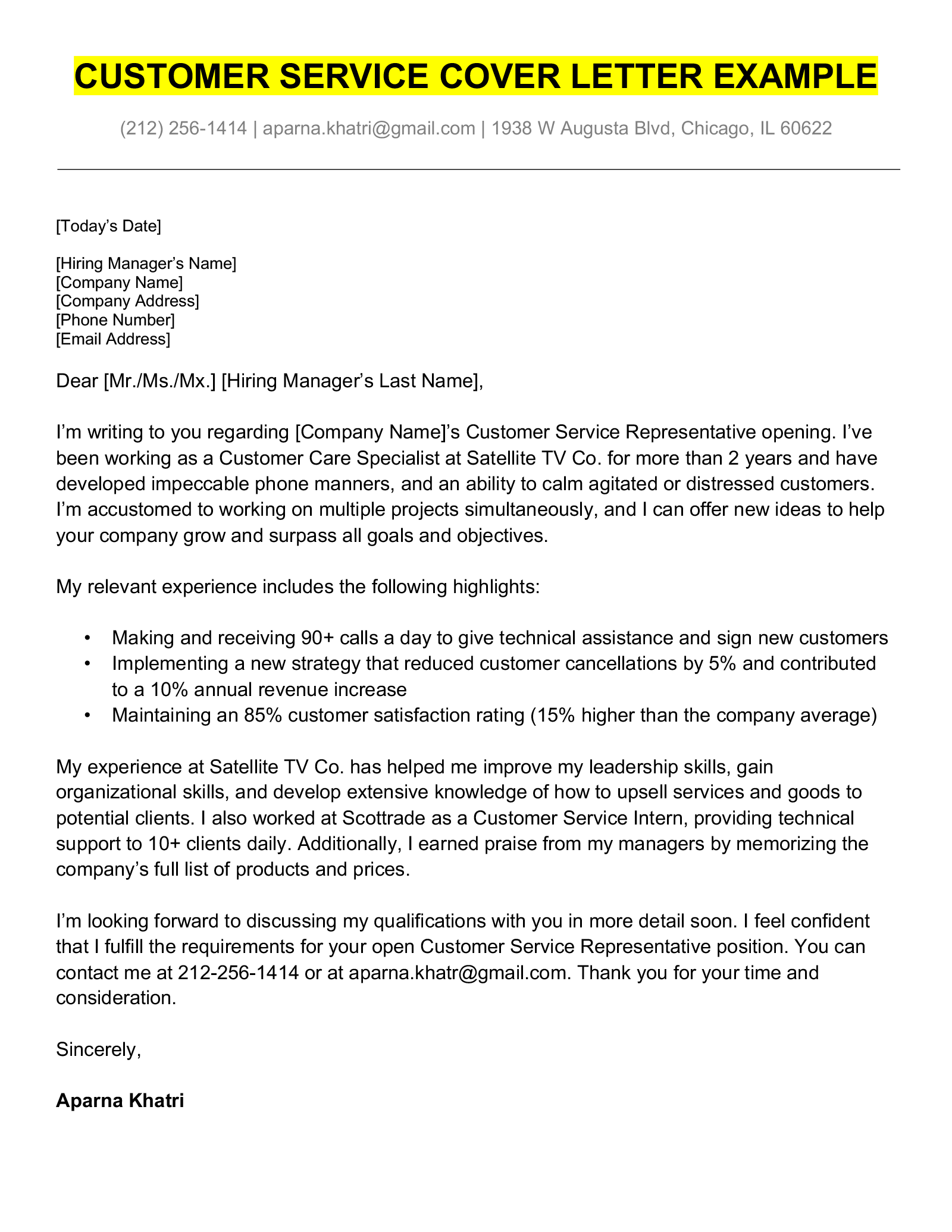The image is an advertisement displaying a customer service cover letter template against a white background. At the top center, there is a yellow highlighted rectangle with black text that reads, "Customer Service Cover Letter Example." Below this header, the top left corner lists placeholders for various details in black text, including "Today's Date," "Hiring Manager's Name," "Company Name," "Company Address," "Phone Number," and "Email Address." 

Following these placeholders, the template continues with "Dear Mr./Ms./Mx. [Hiring Manager's Last Name]," leading into a professionally crafted example that underscores a candidate's experience and skills in customer service. The body of the text details how to write an effective cover letter, mentioning experiences such as working at "Satellite TV Co. for more than two years" and highlighting key abilities like "impeccable phone manners" and the "ability to calm agitated or distressed customers." The letter is formatted into paragraphs, each focusing on different aspects of professional qualifications and personal attributes suitable for a customer service role. The overall style is clean and easy to follow, providing clear placeholders for customization to match the applicant's specific details and the prospective employer.